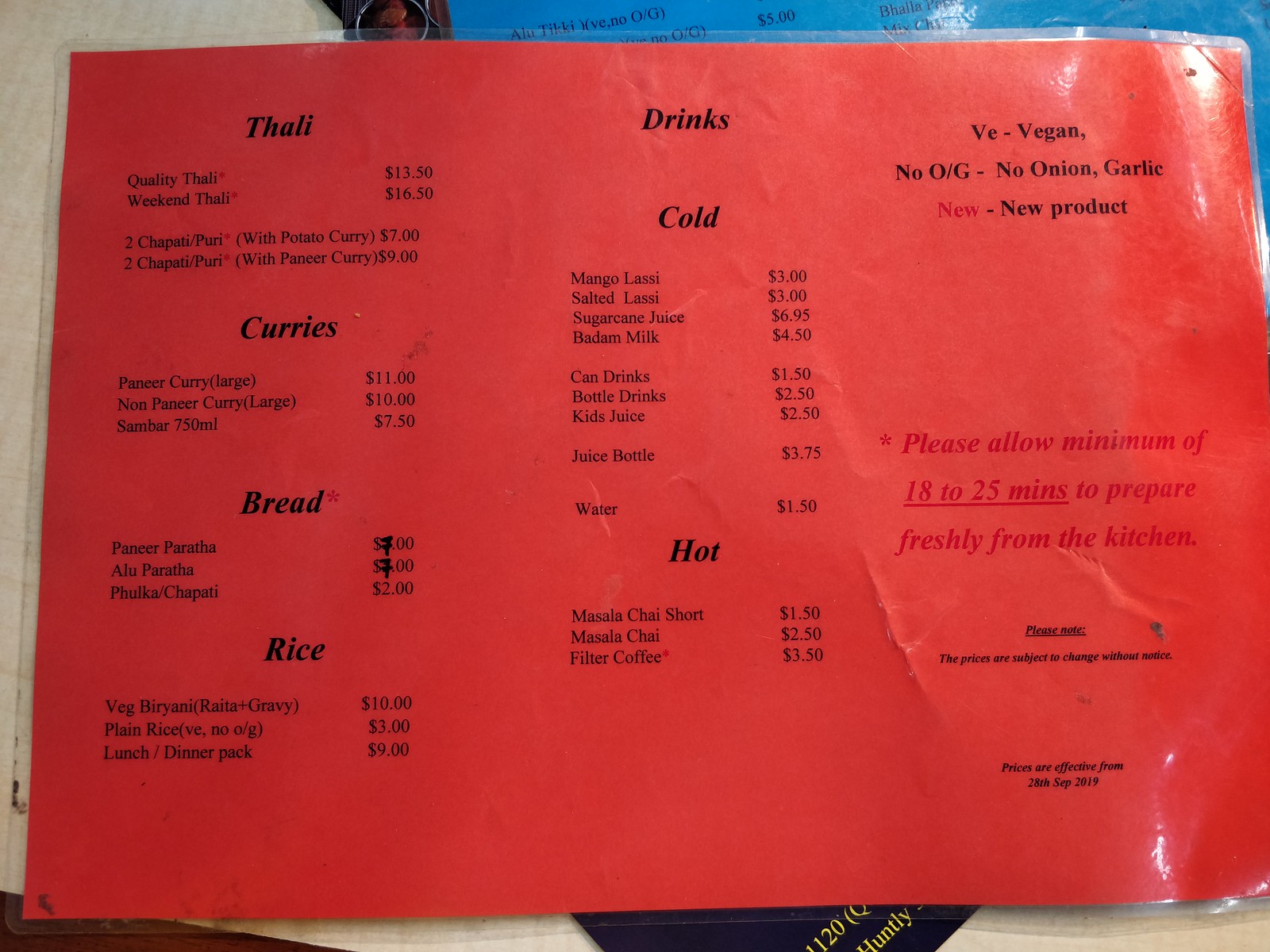This image features a detailed menu of Indian cuisine items. The menu is organized as follows:

**Thali Options:**
- Thali
- Quality Thali
- Weekend Thali

**Bread and Curries:**
- Two Chapati or Puri with Potato Curry or Paneer Curry
- Curries including Pepper Curry, Non-Pepper Curry, and Sambar
- Bread options such as Paneer Paratha and Chapati

**Rice Selections:**
- Vegetable Soup Plate
- Dinner Pack

**Beverages:**
- Mango Lassi
- Salted Lime Tea
- Sugarcane Juice
- Buttermilk
- Canned Drinks
- Bottled Drinks
- Kids' Juice
- Juice Bottles
- Water

**Hot Beverages:**
- Masala Chai (Short)
- Masala Chai
- Filter Coffee

The legend at the bottom provides key dietary symbols:
- V = Vegetarian
- No OG = No Onion or Garlic
- New = New Product

There is also a note indicating that a minimum of 18 to 25 minutes is required to prepare the items freshly in the kitchen.